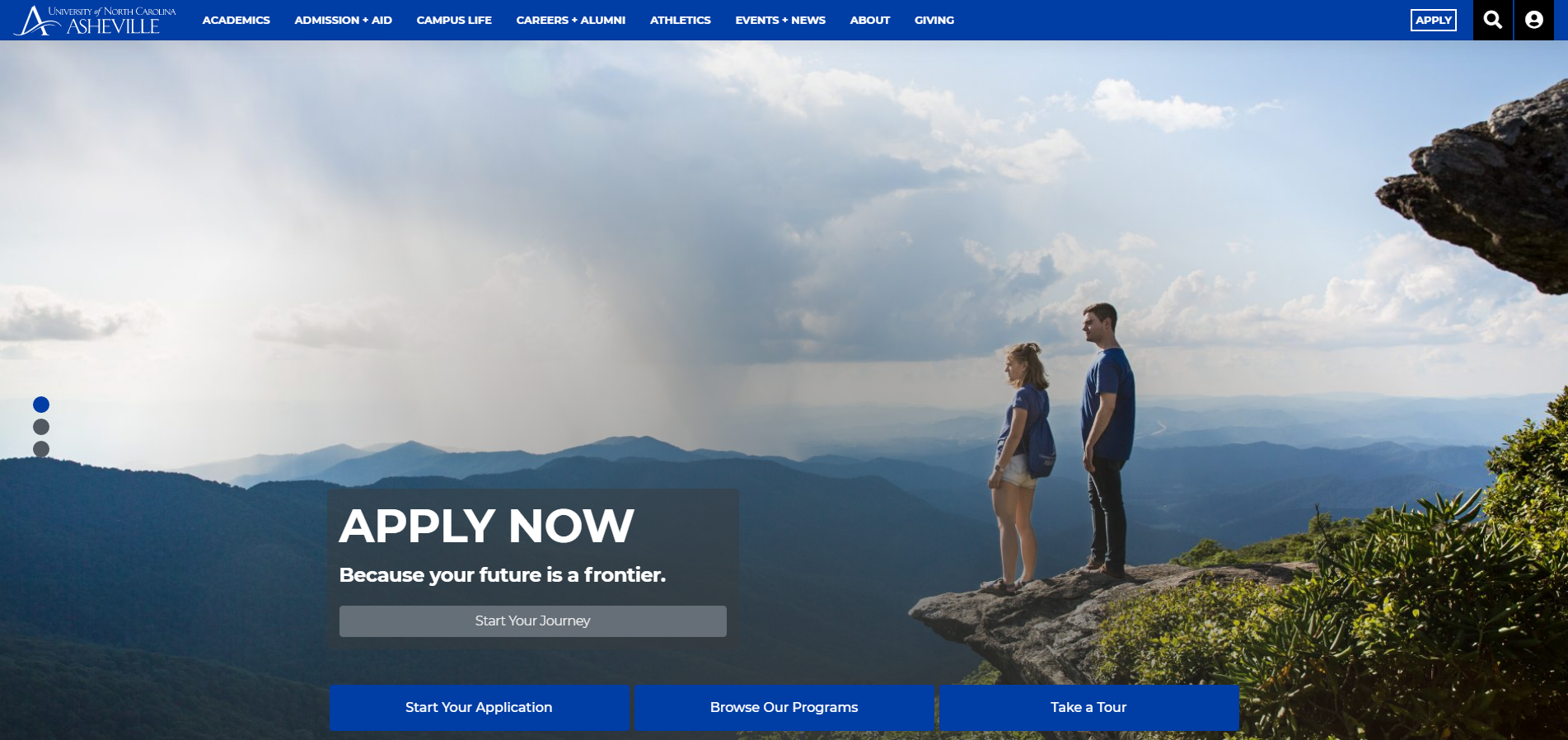Screenshot of the official Asheville website: The left side features the Asheville logo, which depicts a stylized "A" with a unique horizontal line that starts from the left leg of the letter and ascends towards the middle of the right leg. Positioned above the logo, within a blue horizontal bar stretching across the top of the screen, are the words "University of North Carolina". To the right of the logo is the website's main menu, including the following tabs: Academics, Admission & Aid, Campus Life, Careers & Alumni, Athletics, Events & News, About, and Giving. In the background of the site, there are two individuals standing at the edge of a scenic mountain, gazing into the sky.